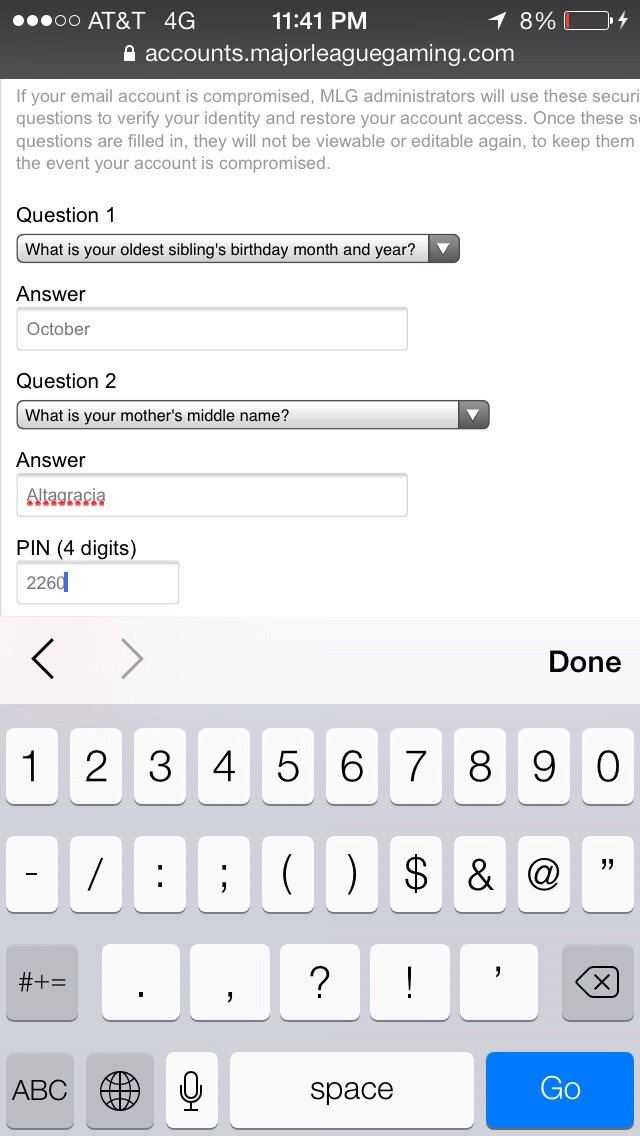This is a detailed screenshot from a smartphone displaying the process of setting up account recovery options on accounts.majorleaguegaming.com. At the top, the status bar shows the phone is connected to AT&T's 4G network, it's 11:41 p.m., and the device has an 8% battery charge. Below this, there's a grey banner with a white padlock icon next to the website URL, indicating it's a secure site.

A grey-background column of text explains that if the user's email account is compromised, MLG administrators will use the provided security questions to verify identity and restore access. These secret questions, once filled, cannot be viewed or edited again.

The security setup includes two secret questions and a PIN. The first question asks for the oldest sibling's birthday month and year, to which the user has responded with "October." The second question inquires about the user's mother’s maiden name, answered with "Alta Gracia." Finally, the user has created a four-digit PIN, "2260."

At the bottom of the screen, the phone's numeric keypad is visible, suggesting the user is in the process of entering or has just finished entering the PIN. The entire setting reflects the measures taken to secure access to the user's account in case of email compromise.